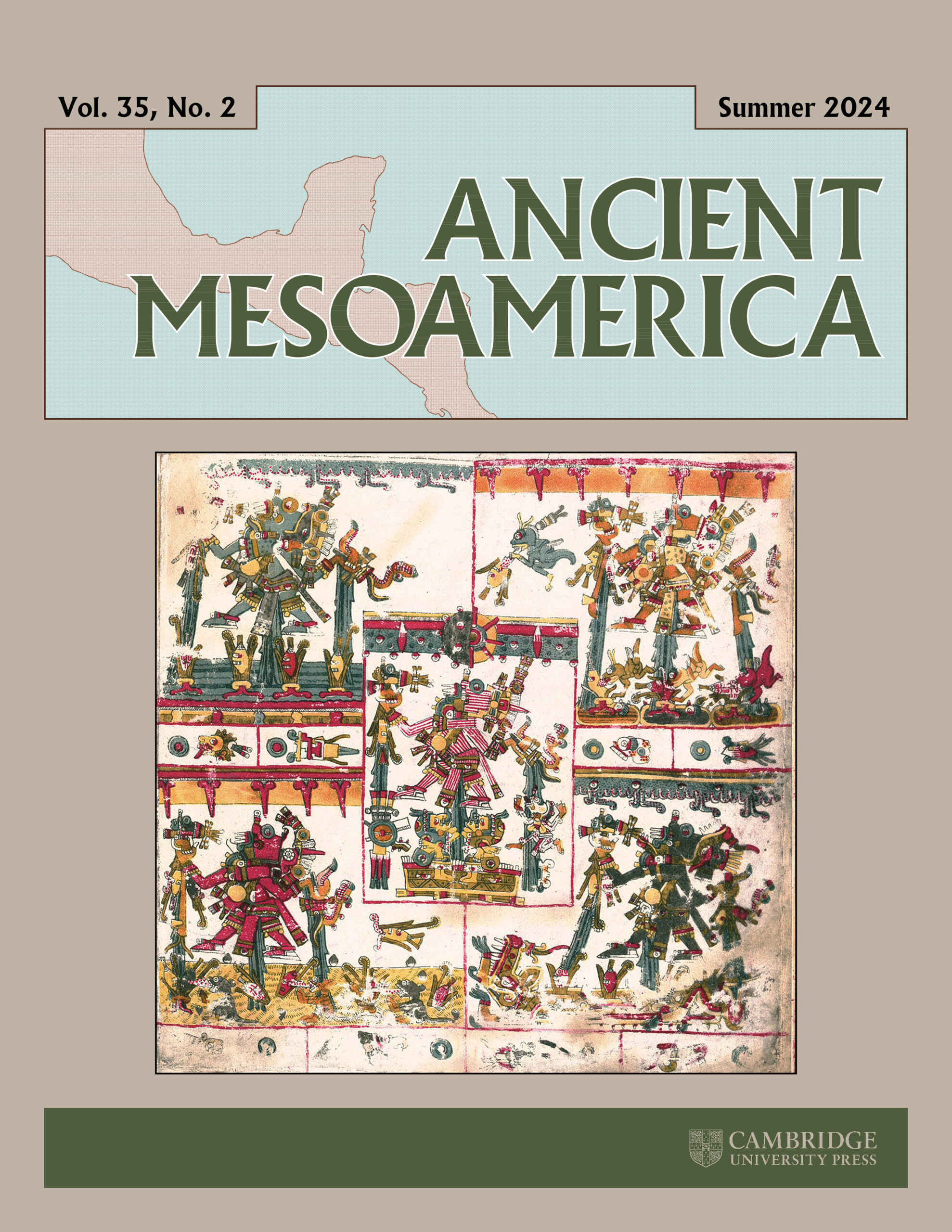The cover of the book or magazine titled "Ancient Mesoamerica," Volume 35, Number 1, Spring 2024, features a central illustration of a golden disc with red and grey accents. The disc's design is abstract and possibly includes hieroglyphic-like elements. Below the illustration, the text "5 centimeters" is displayed, indicating a scale. The central image is set against a grey background, framed by a larger bluish-pink backdrop. A label at the top prominently displays the title "Ancient Mesoamerica" in a large font. In the bottom section, a green bar spans horizontally, featuring a crest logo of a shield and the text "Cambridge University Press." The overall cover design suggests a scholarly publication focusing on artifacts and historical themes.